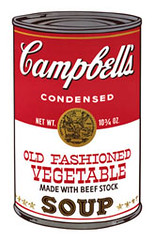This highly detailed, color illustration captures a can of Campbell's Old-Fashioned Vegetable Soup, clearly inspired by Andy Warhol's iconic pop art style. The top portion of the label is a vivid red with "Campbell's" elegantly scripted in white followed by "Condensed." The red background transitions into a white lower half where "Old-Fashioned Vegetable Made with Beef Stock" is written in red and black lettering. Dominating the lower white area, the word "SOUP" is displayed prominently in large black letters, flanked by four golden stars on each side. A distinctive gold seal or crest divides the red and white sections at the center of the can, adding an air of traditional craftsmanship though its details are somewhat indiscernible. The can itself retains realistic metallic features at the top and bottom, reinforcing the illusion of depth and texture against the stark white background where it stands out. The overall effect is a classic, yet modernized homage to the familiar Campbell's soup can, celebrating its place in both art and popular culture.